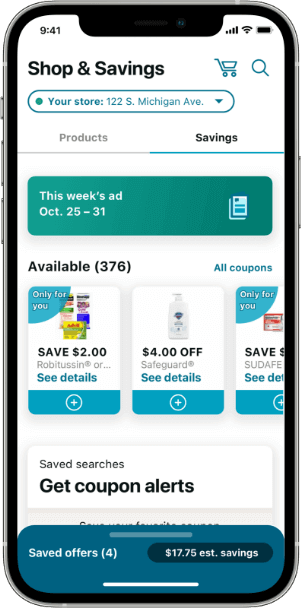This image is a detailed screenshot of a smartphone displaying an app likely related to shopping or savings. The entire phone, including its gray edge housing, is visible.

On the left-hand side of the phone, there are three buttons, and on the right-hand side, there's one gray button. The screen shows a white background. At the top left corner, the time reads "9:41" in black, and at the top right, there are four black Wi-Fi bars alongside a full black battery icon.

Prominently, at the top of the screen in bold black lettering, it says "Shop and Savings." To the right of this text, there are two icons: a blue shopping cart and a blue magnifying glass, indicating search functionality. Below this, there's a blue-outlined oval bar with blue text in the center that reads "Your Store 122 South Michigan Avenue," accompanied by a blue down arrow for a dropdown menu.

Underneath this bar, there are two tabs. On the left, in gray text, it says "Products," and on the right, in bold black text it says "Savings," which is currently selected as indicated by a blue underline.

Below these tabs is a rectangular blue bar with white lettering. The text on the left reads "This Week's Ad October 25th through 31st," and on the right, there is a small icon of a document.

At the bottom portion of the screen, text reads "Available 376" in black, indicating the number of available coupons, and "All Coupons" on the right. Below this line, there are visible coupons:

1. On the left, a $2 coupon for Robitussin with a blue "See details" link and a blue bar at the bottom featuring a white circle with a plus sign for adding the coupon.
2. In the center, a $4 coupon for Safeguard, similarly formatted with the "See details" link and the blue bar with the add option.
3. On the right, a partially visible coupon for Sudafed, also formatted alike.

Beneath these coupons is a white rectangle with the text. In gray, it says "Save searches," followed by "Get coupon alerts" in bold black.

At the very bottom of the app, there's another blue oval bar with a lighter blue line at the top and a white line at the bottom, both centered. On the left side, in white text, it says "Saved Offers (4)," indicating the user has four saved offers. On the right side, against a darker blue or black background, it reads "1775" in white, representing the estimated savings amount.